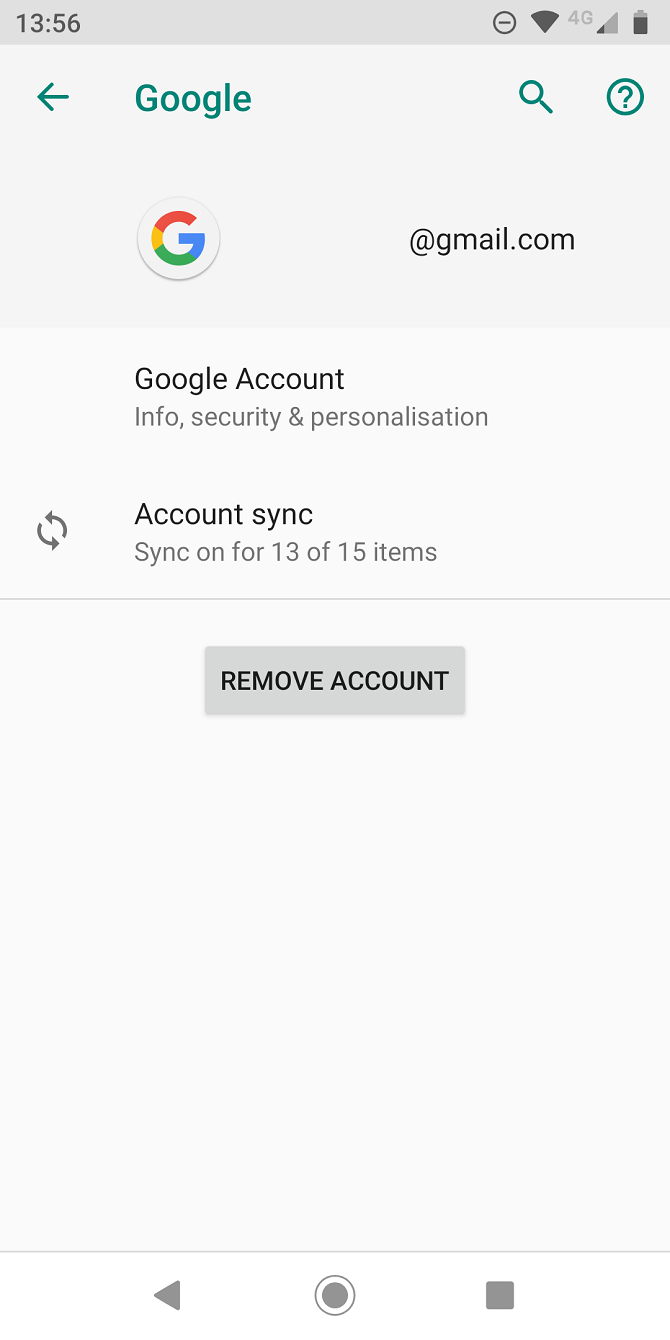A screenshot captured on an Android device showcases the Google app interface as the user navigates through the process of signing into their Google account, specifically for Gmail. Upon successful login, the user is presented with a set of account settings. 

The first setting option, labeled "Google Account," allows access to further configurations related to account security and personalization. The second setting option provides synchronization controls, indicating that 13 out of 15 items are currently set to sync, with additional options available to sync the remaining items.

Near the bottom of the screen, there is a conspicuous grey rectangular box offering the option to remove the account entirely. The interface also includes standard navigation buttons: a circular home button at the center, a grey square representing recent apps on the bottom right, and a grey triangular back button on the bottom left.